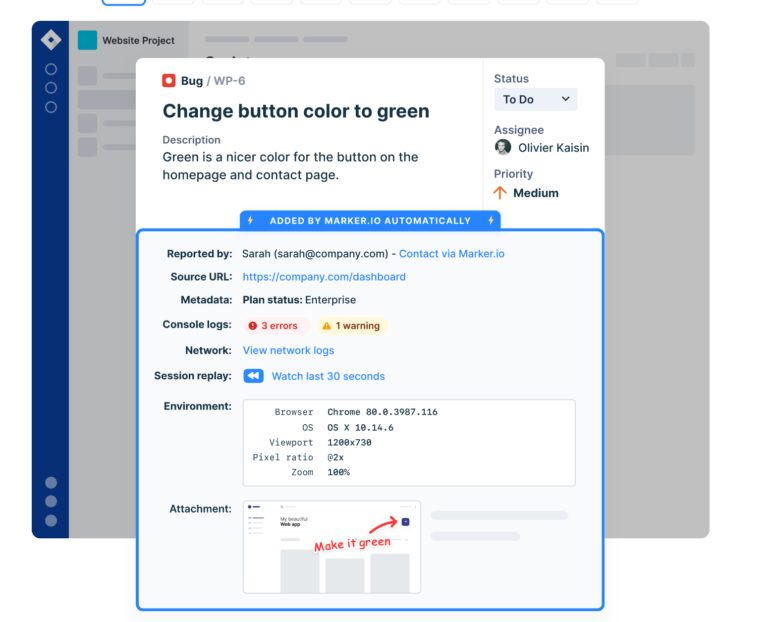Detailed Caption:

This is a screenshot of a web application displaying a simple webpage with a gray filter overlay. The background webpage features a clean, white design with the title "Website Project" prominently displayed at the top in black font. On the left side, a long horizontal blue bar is visible.

The focal point of the screenshot is a pop-up menu centered on the screen, obscuring part of the grayed-out webpage behind it. The pop-up menu has a white background and is bordered delicately, adding to its simplicity. At the top, "Bug/" is written in black font, followed by "WP-6" in gray font.

Below the header, the main text in black font reads, "Change button color to green." Beneath this instruction, a description in gray font states, "Green is a nicer color for the button on the home page and contact page."

To the right side of the pop-up menu are several fields:

- At the top, "Status" is written in gray font next to a gray drop-down menu, which currently displays "To Do" in black font.
- Below the status field, "Assignee" is labeled in gray font next to a small profile picture of a white man, with the name "Olivia Kaysen" in black font beside it.
- Further down, "Priority" is marked in gray font, with the priority level noted as "Medium" in black font.